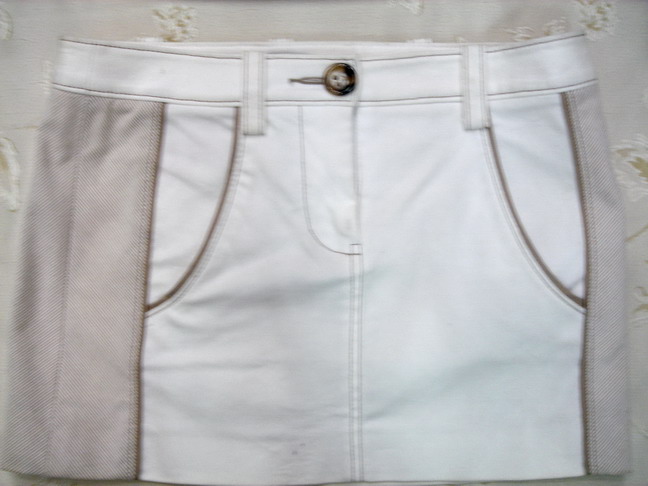The photograph showcases a white clothing item that could either be a pair of shorts or a miniskirt, lying flat on a floral-patterned cloth. The garment is predominantly white, featuring a combination of jean-like material and striped fabric. It is accented with light brown and dark brown details, including very thin brown borders along the seams and pocket edges. The waistband is about an inch and a half wide and includes a couple of white belt loops. A notable feature is the large brown button at the center, which has a bit of black pigmentation. The garment appears to have a folded top edge, revealing its hem, and is intricately sewn with a double layer of stitches. The sides of the item, around the hips, feature light brown and dark brown hues that blend into the overall design.